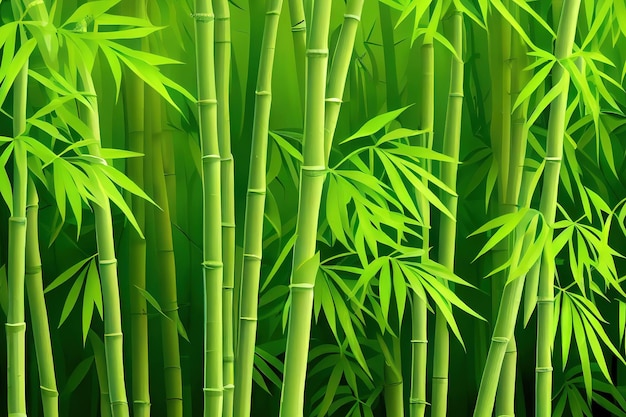A close-up, digitally enhanced image showcases several bamboo-like stalks and stems, characterized by segmented sections occurring every six to seven inches. These stalks vary in hues from light green to a yellowish tint. Delicate, thin leaves, predominantly curving to the right but some to the left, adorn each stalk, with each stalk having five to eight leaves each. The foreground is dense with these stalks, each approximately two inches in diameter, while the background reveals more foliage in a darker green, evoking a jungle-like setting. The overall effect is serene and meticulously curated, akin to a high-quality poster or computer screensaver designed to provide a calming visual experience.